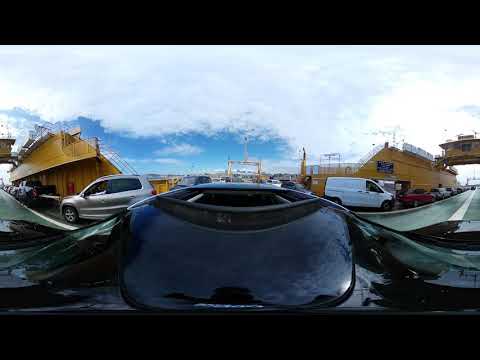The image captures a bustling industrial dock area from a high vantage point, showcasing a 360-degree view. The setting is outdoors and appears to be taken during the day under partly cloudy skies, allowing for ample natural light. The foreground prominently features a variety of parked vehicles, including a silver SUV, black pickup truck, white van, and a red vehicle, among others, positioned along a street lined with long wooden buildings with walkways. These buildings and the vehicles are central to the composition. In the midground, an industrial crane stands out, hinting at the dock's shipbuilding operations. Beyond the street, the edges of the water are visible, with additional cranes punctuating the skyline, reinforcing the industrial atmosphere. The scene is framed by a solid black border at the top and bottom, and the overall color palette includes hues of black, white, gray, blue, red, brown, tan, and green. The image is both detailed and dynamic, with a clear indication of the various elements that make up this busy dockside environment.